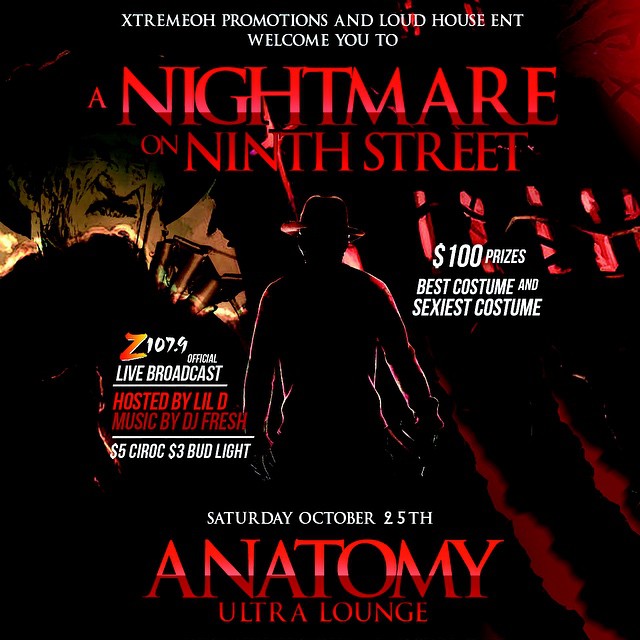This image is a partial view of a promotional poster for an event called "A Nightmare on 9th Street," organized by Extremio Promotions and Loud House Entertainment. The poster features a bold, attention-grabbing design with a black background, red, and white text. Central to the image is a man wearing a hat. The text details various elements of the event, including a $100 prize for the best costume and sexiest costume. Additionally, it advertises Z107.9's official live broadcast hosted by Lil D, with music by DJ Fresh. The event takes place on Saturday, October 25th at the Anatomy Ultra Lounge.